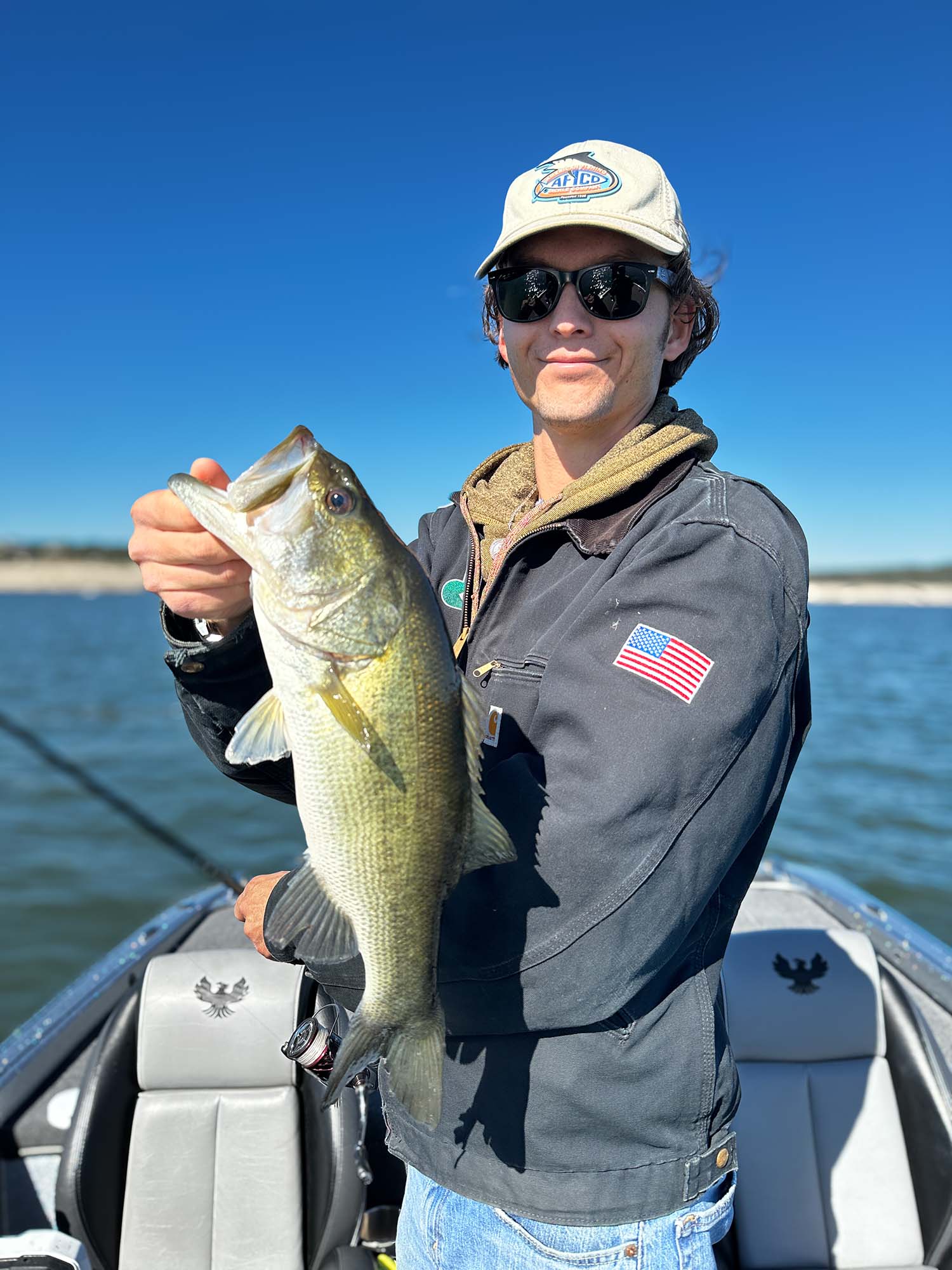Standing on a two-person boat, a young white male in his early 20s is proudly displaying his recent catch, an 18-inch bluish-green fish, possibly a bass, held vertically by its mouth in his right hand. Clad in a layered outfit consisting of a dark blue jean jacket with an American flag patch on the left shoulder, a brown hoodie underneath, and a shirt, he pairs it with light blue jeans. His attire is complemented by black Wayfarer-style sunglasses and a white fishing cap emblazoned with the logo "AFCO" and a fish emblem. His curly brown hair peeks out from under the hat, and he's beaming with a broad smile. In his left hand, he holds a slightly out-of-focus fishing rod. The boat, equipped with gray leather seats featuring a gold eagle stitched into the headrest, is either on the ocean or a lake, as evidenced by the distant strip of beach sand. The open water and serene background highlight the triumph of his fishing adventure.